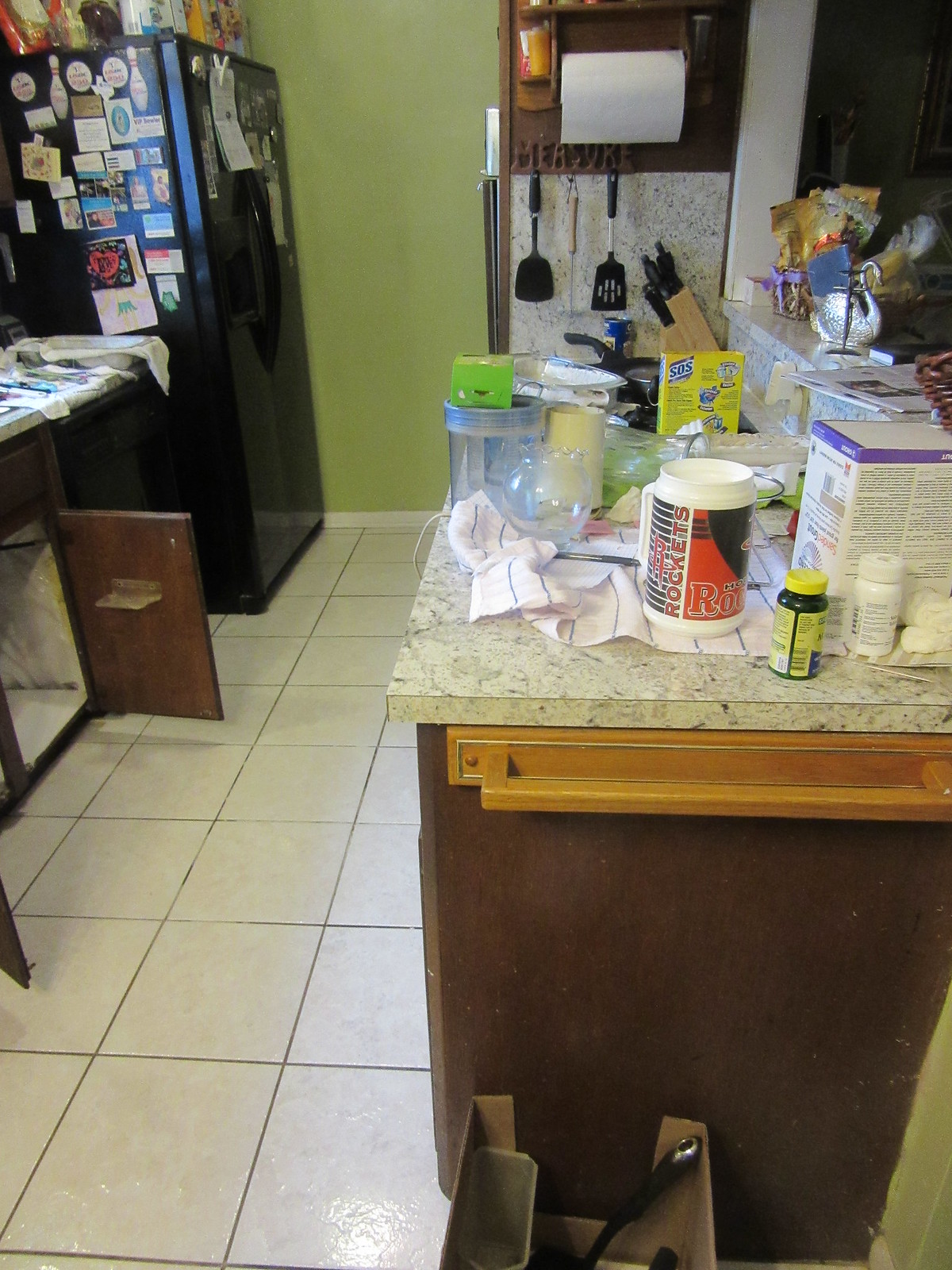This photograph depicts a bustling kitchen scene. On the left side of the image, there is a black refrigerator adorned with an assortment of magnets and business cards primarily on its side, while the front features a large piece of paper clipped to it with visible handwriting. Atop the refrigerator sit various food items, including cereal boxes and other packages. Below, an open brown cabinet, part of a larger kitchen unit, reveals itself alongside a counter draped with fabric items.

Dominating the right-hand side of the image is a spacious counter surface, cluttered with vitamin bottles, a box of SOS pads, and a long dish towel or cloth. Additionally, an open cup or package labeled "Rockets" and a large white box with purple accents catch the eye. Hanging above the counter are kitchen tools, including two spatulas and another utensil. Completing the scene is a swan figurine and a roll of paper towels, adding a touch of personality to the kitchen space.